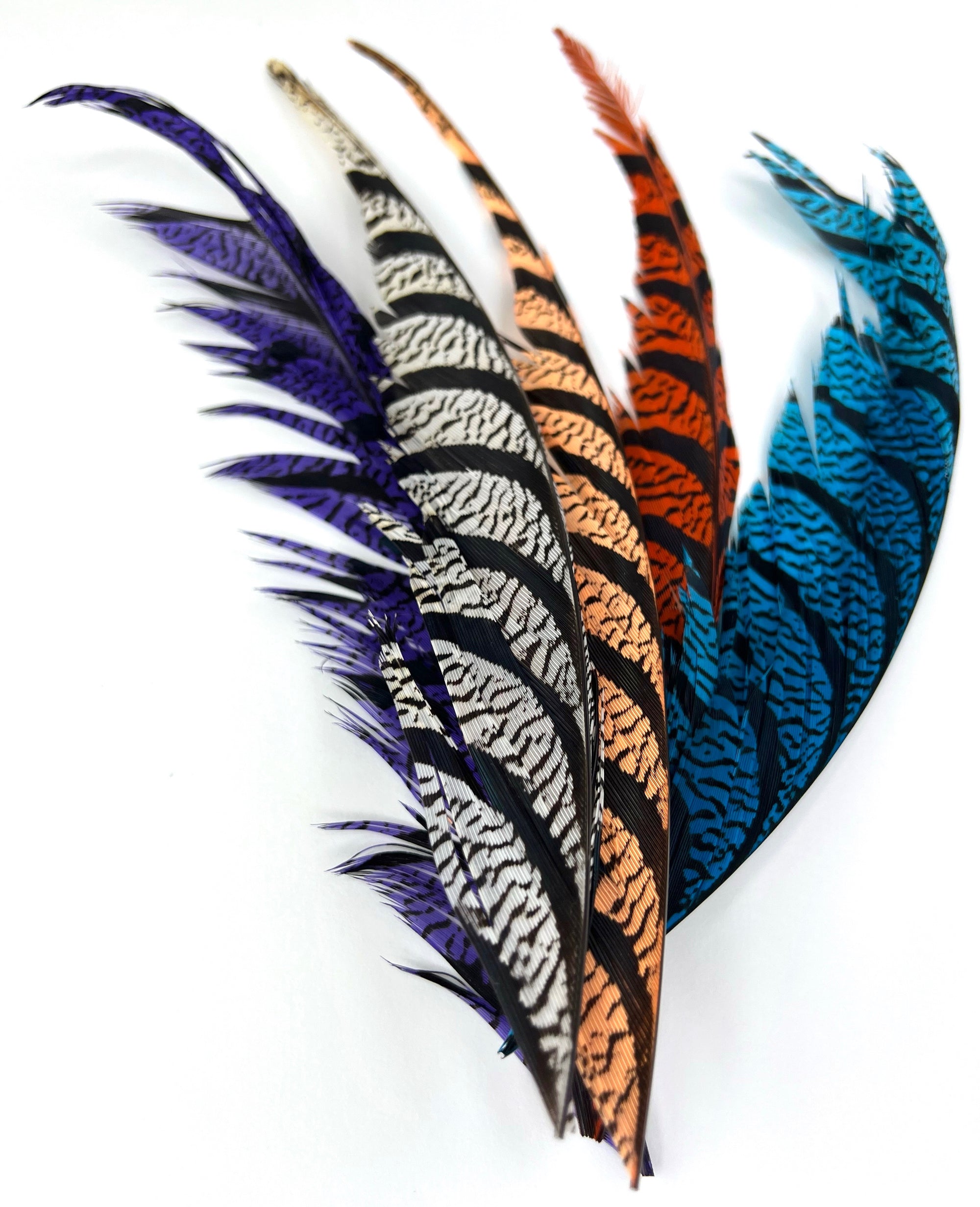The image depicts a vivid collection of five feathers, each standing upright. The sequence showcases diverse, striking colors: starting from the left, there's a feather with deep purple hues, followed by a pristine white one adorned with a singular black stripe. Next is an orange feather, similarly marked with black, succeeded by a vibrant red feather featuring the same black stripe pattern. Completing the row on the far right is a turquoise feather, also highlighted with a distinct black stripe. All the feathers share a consistent design of thick black stripes, complemented by small, intricate squiggly black lines among them, enhancing their visual intricacy and unity despite the varied colors.